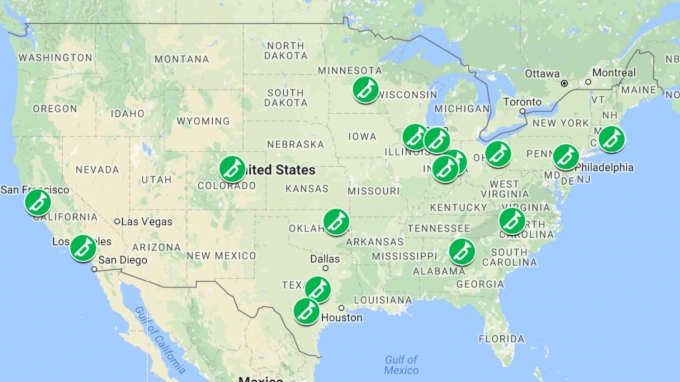This image depicts a detailed and expansive map of the United States of America. The rectangular map showcases the entire country, stretching down to include the Gulf of California and the Gulf of Mexico, which extends beneath one of the islands off the coast of Florida. On the northern edge, the map almost touches the border with Canada, dipping into the Great Lakes region, and highlights Canadian cities such as Toronto, Ottawa, and Montreal, though some city names are partially obscured.

Distinctive green circles with white trumpets, encircled by a white border, are strategically placed across various locations on the map, presumably indicating significant sites related to trumpets or music. These circles can be found in:

- San Francisco and either Los Angeles or San Diego in California.
- An unspecified location in Colorado.
- Minnesota.
- Two locations in Wisconsin.
- Two locations in Indiana.
- Oklahoma.
- Two locations in Texas.
- North and South Carolina.
- Pennsylvania.
- New Jersey.
- Connecticut.
- Massachusetts.

Virginia does not feature any of these marked sites. The exact purpose of these trumpet symbols remains unclear from the description.